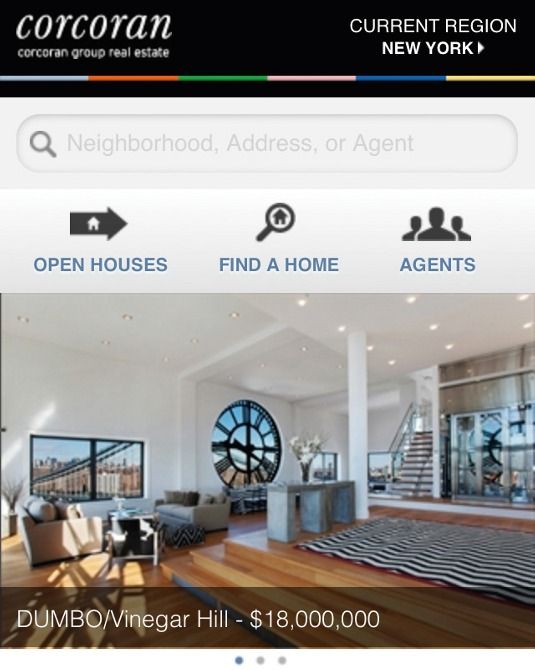The image shows a screen capture from a smartphone, displaying a sleek and modern interface from the Corcoran Group Real Estate website. The brand name "Corcoran" is prominently featured at the top in elegant, lowercase lettering with a slight flourish at the tail ends, set against a stark black background. To the right of the logo, the text "current region: New York" is accompanied by a rightward-pointing arrow.

Below this header, a horizontal bar transitions through several colors—starting with gray, followed by orange, green, pink, blue, and yellow—creating a visually appealing divider. Beneath the colorful bar, a search section is visible, featuring a magnifying glass icon next to the placeholder text "neighborhood, address, or agent."

Further down, three clickable options are displayed: "Open Houses" indicated by a right-pointing arrow, "Find a Home" with a magnifying glass icon, and "Agents" represented by silhouettes of people.

At the bottom of the screen, a highlighted listing reads "Dumbo / Vinegar Hill" with a staggering price tag of $18 million. The accompanying image showcases a luxurious house with impressive lighting, a clock embedded in the wall designed like windows, and other opulent features, exuding a sense of high-end living and sophistication.